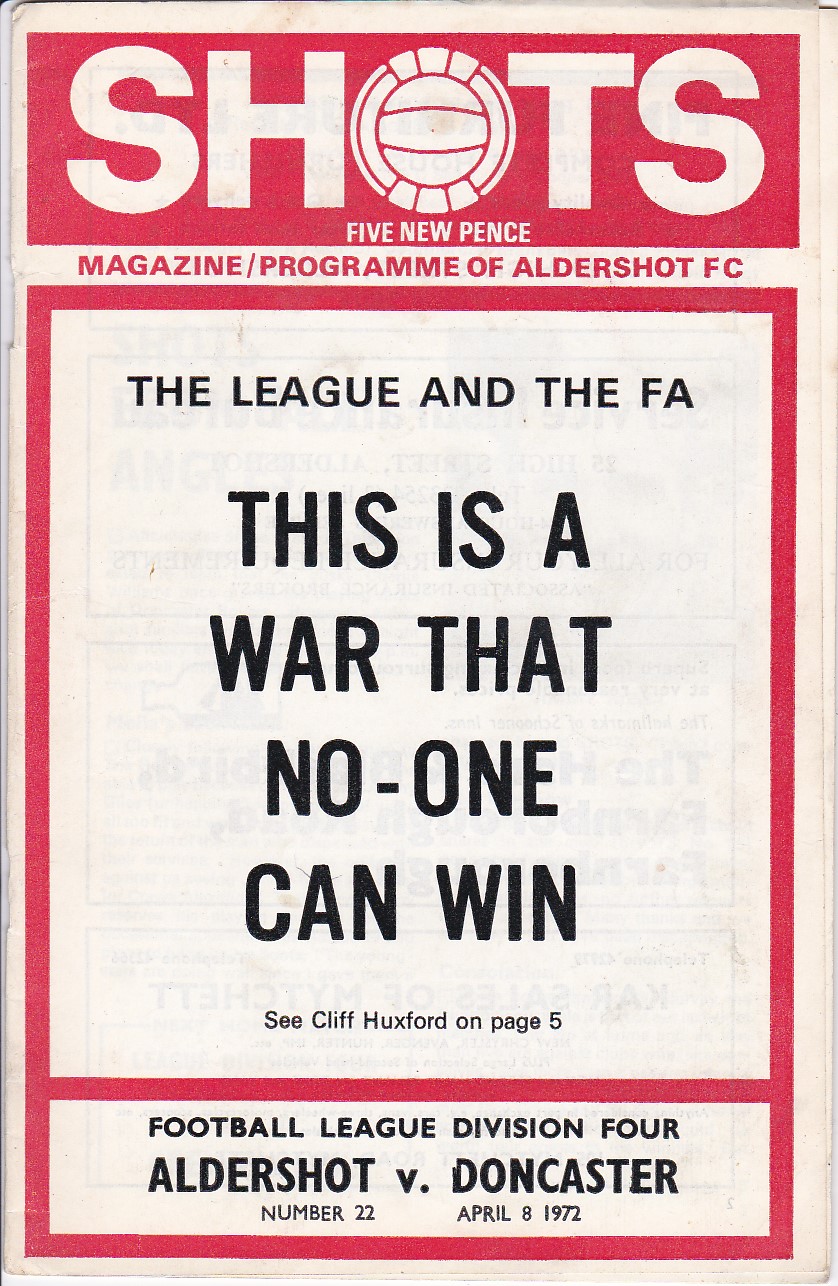This image features the cover of a football (soccer) program magazine predominantly designed in black and red print on a white background. At the very top, there is a red rectangle with white text that reads "SHOTS," where the "O" interestingly resembles a sports ball. Beneath this, in red text against a white background, it states "Magazine Program of Aldershot FC," followed by another prominent red rectangle outline. Inside this outline, in black text, it reads "The League in the FA. This is a war that no one can win. See Cliff Huxford on page 5." Lower down, there's a red line separating more black text that says "Football League Division 4 Aldershot v. Doncaster, Number 22, April 8, 1972." The cover's color scheme is a striking mix of red and white with black text, creating a bold visual contrast.